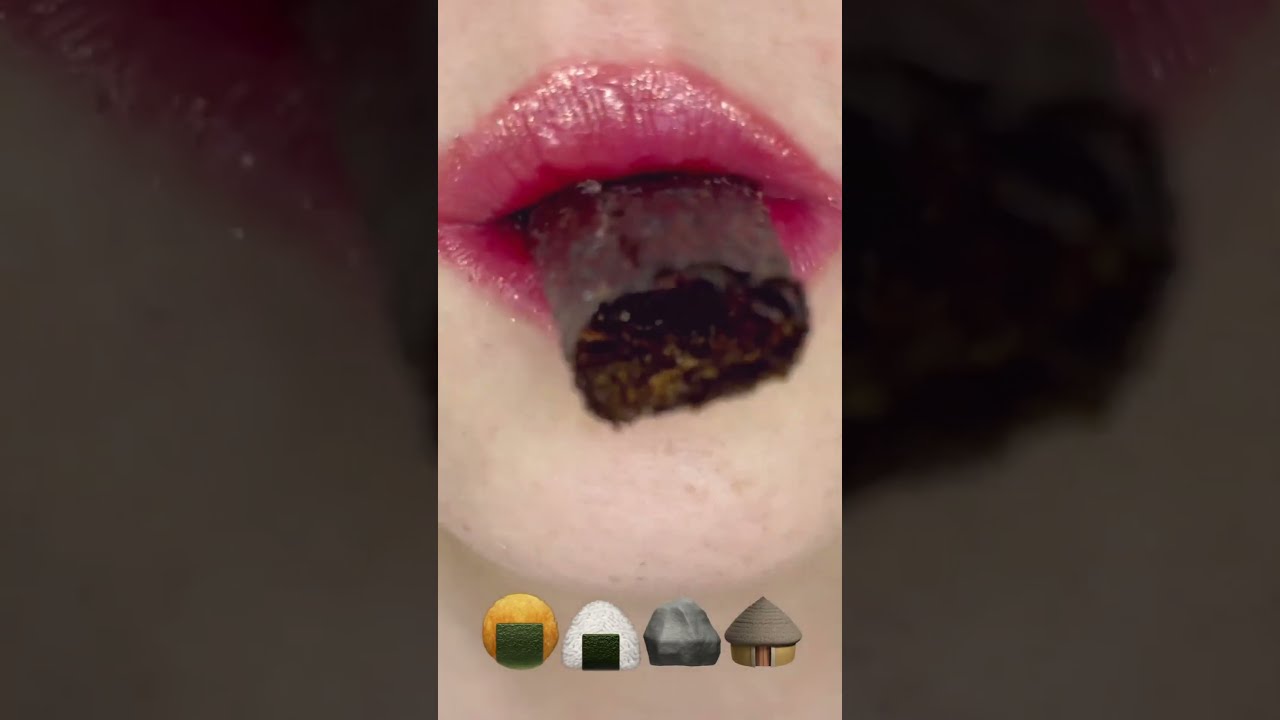The image features a close-up selfie of a light-skinned woman's mouth, accentuated with glossy, vibrant pink lipstick, and slightly zoomed in to include parts of her chin. In her mouth, she holds a brown, cylindrical object that resembles either a cigar, taffy, or possibly a Slim Jim. Flanking the central image are larger, rectangular, zoomed-in sections of her lips, highlighting their shine and rich color, set against a stark, dark background.

Below this central image, a row of four small emojis is visible, each depicting distinctly different 3D objects: a circular food item wrapped with green seaweed, a triangular rice ball also adorned with seaweed (resembling typical Japanese onigiri), a gray stone or boulder, and a beige, straw-roofed hut, suggestive of a traditional tribal structure.

This detailed description combines and emphasizes the repeated elements of the image and the distinctive features highlighted by each observer.